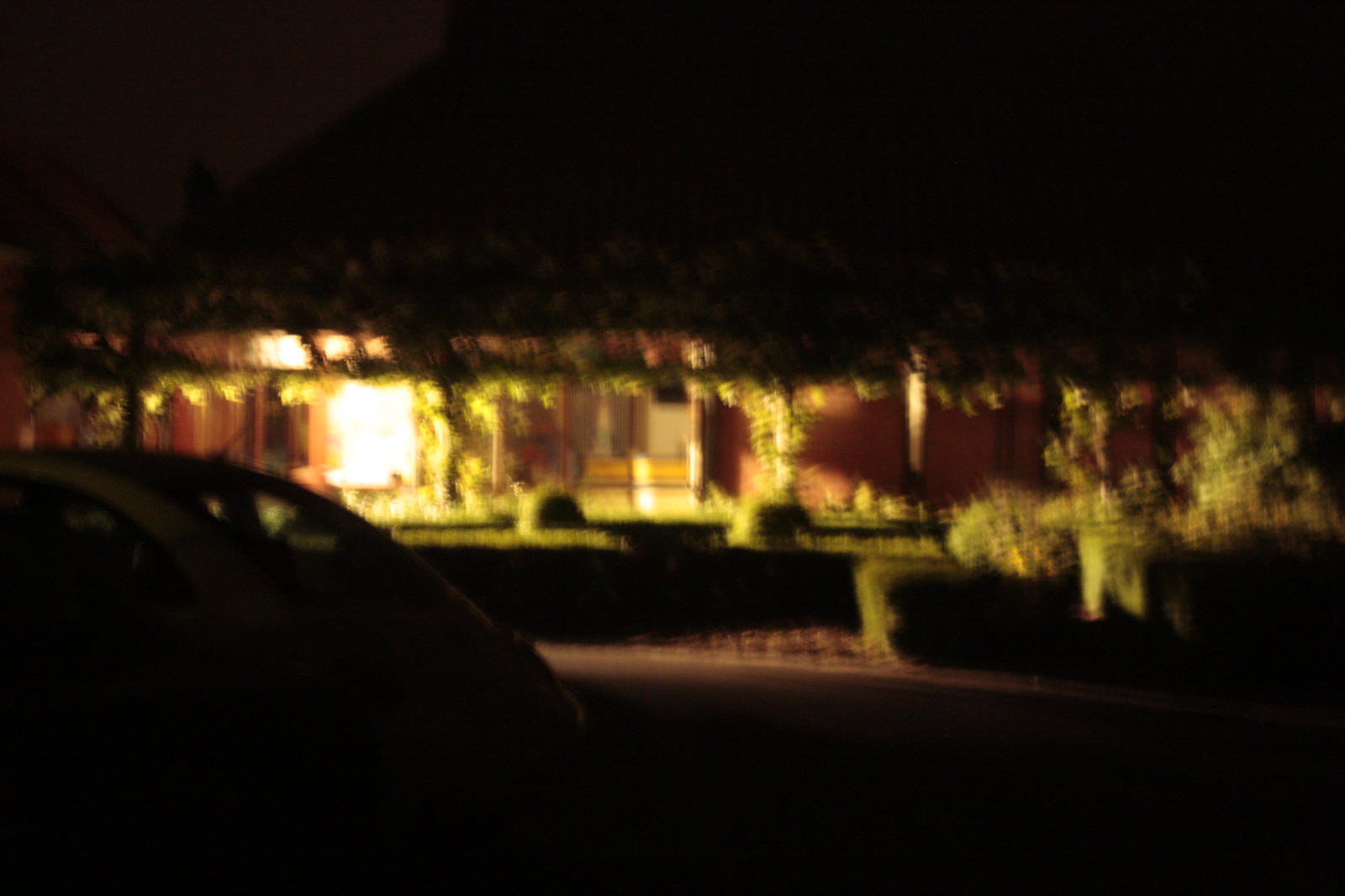This photograph captures a nighttime scene at the front of a house, enveloped in darkness with only a bright porch light illuminating the area. The image quality is fairly low, adding to the obscurity. On the lower left side, a silhouette of a car, likely a Volkswagen Beetle based on its curved shape and visible radio antenna, is just discernible. The house features a large porch supported by several beams, many of which are wrapped in vines extending to the roof, adding a leafy texture to the structure. Surrounding the porch are numerous plants and recently trimmed bushes. The faint outlines of windows are visible; one appears to have curtains. The scene is predominantly black due to the lack of ambient light, making specific colors indiscernible except for the intense glow from the porch light that overshadows its immediate surroundings.